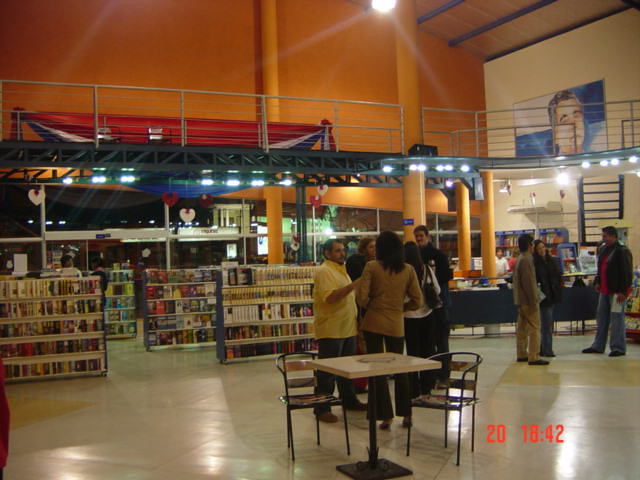The image captures the lively common area of a combined bookstore and media store, featuring a mix of industrial and artistic design elements. The open space in the foreground has a white tile floor and is furnished with tables and chairs, where people are casually conversing in small groups. In the background, there are shelves filled with books and possibly video cassettes, further suggesting the dual nature of the store. Colorful walls—orange at the back and beige on the right—frame the space, adorned with artwork, including a blue and white painting of a man. A staircase in the right part of the image leads up to a second story balcony that overlooks the seating area below. The aesthetic blends industrial girders with vibrant decorations, including a red, white, and blue banner on the orange wall. The lower right corner of the image bears the timestamp "2018:42," indicating the possible date and time the photo was taken.